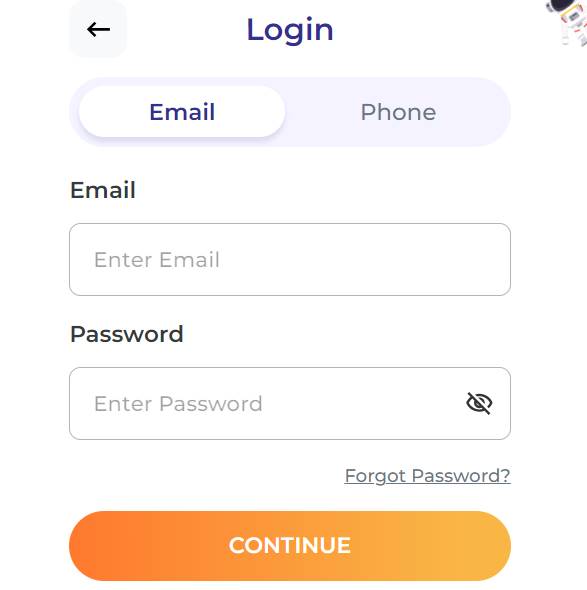This screenshot showcases a zoomed-in view of a login page, which could belong to either a mobile app or a web page, making it difficult to definitively identify the platform. The layout is in portrait orientation, which suggests it might be for mobile, but the zoomed-in perspective leaves room for ambiguity.

In the top left corner, there is a "Login" button or touch area. The central part of the interface features a stylish, darker gray section with inputs for login credentials. These inputs, labeled "Email" and "Phone," rest against a light gray background over a predominantly white interface.

The "Email" field, currently selected, is accentuated with a highlighted border, containing a prompt for the user to "Enter email." Below it, the "Password" field also invites the user to "Enter password," accompanied by an eye icon that allows toggling the visibility of the entered password—a handy feature to avoid input mistakes.

Below the password field, there's a "Forgot password?" link, underlined in gray for easy identification, enabling users to reset their password if needed. At the bottom of the page is a prominent orange "Continue" button, completing the minimalistic and modern aesthetic of the login page.